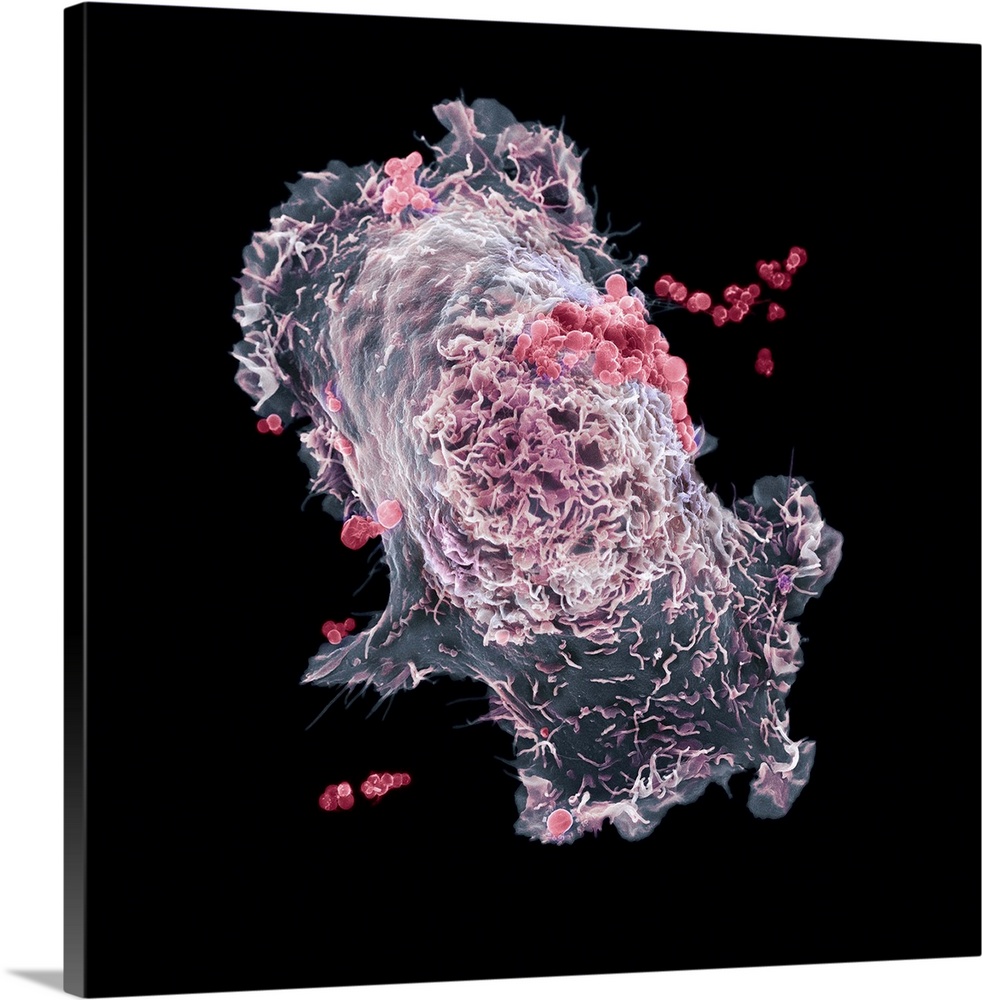The image appears to be an intricate piece of abstract art, centrally positioned on a square black canvas. The artwork, which has the texture reminiscent of jellyfish but not their shape, showcases a complex combination of colors including vivid pinks, reds, whites, grays, and shades of purple. This digital creation, possibly depicting a living organism or molecular structure, features a chaotic and textured central form that might be slimy, surrounded by numerous red, circular elements resembling red blood cells. The black canvas provides a stark contrast, accentuating the striking and immersive visual chaos of the vibrant colors and forms within the piece.